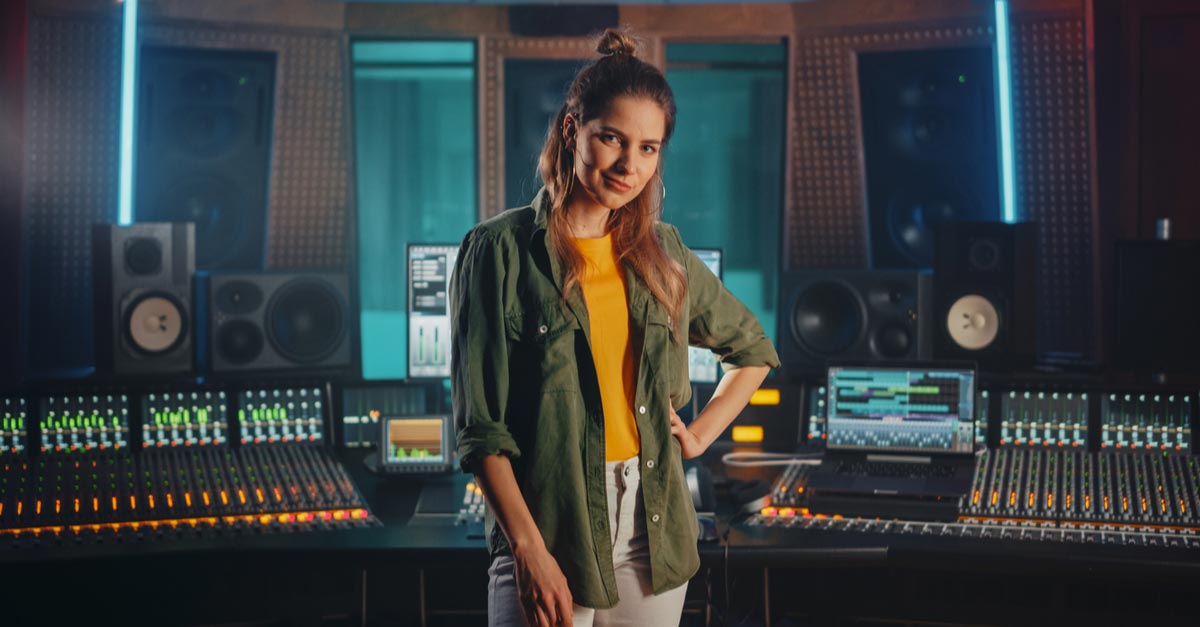The image appears to be an AI-generated rendition of a recording studio scene, featuring a woman standing centrally. She has light skin, long hair styled with the top half in a bun, and is dressed in a khaki green button-down shirt with the sleeves rolled up to her elbows, exposing an orange shirt underneath. She pairs this with white jeans. Her left hand rests on her hip while her right arm hangs loosely, though her right hand appears unnaturally enlarged and her fingers deformed. The studio setting is detailed with multiple black speakers flanking the scene on both sides, a plethora of music equipment including control panels with sliders and buttons, and a laptop displaying music software positioned to her left. Blue lights decorate the wall behind her, which also features rectangular windows and transparent glass, casting a darker ambiance over the room. The woman's subtle smirk adds to her slightly artificial demeanor within the detailed backdrop of mixers, screens, and other electronic recording devices.